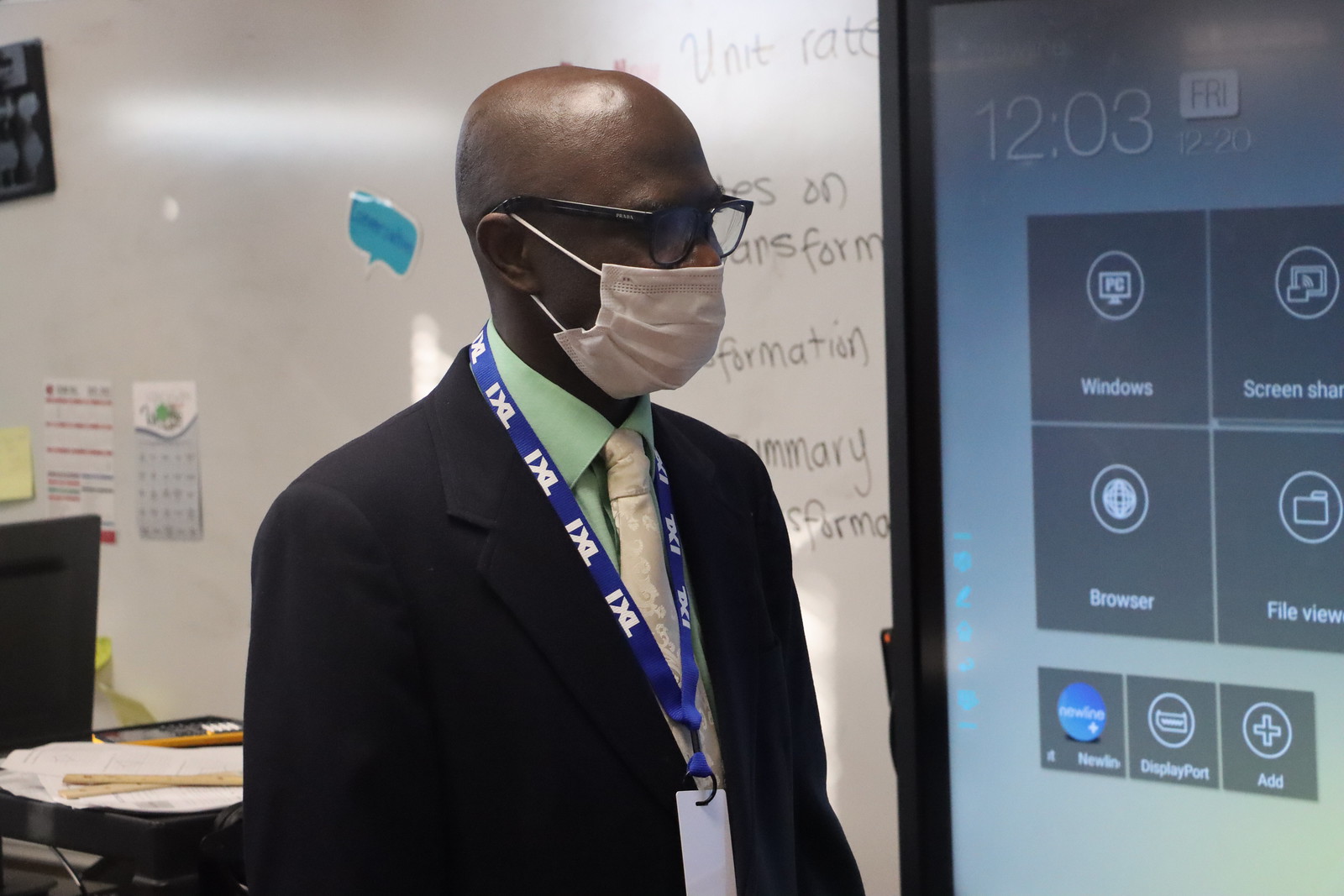The image displays an African-American man, bald, wearing black glasses and a white COVID mask, facing approximately towards the three to four o'clock position. He is dressed in a black suit coat over a green dress shirt, paired with an off-white tie that features a subtle design. Around his neck, he wears a blue lanyard with a tag that is flipped backwards, making it unreadable.

In the background behind the man, there's an off-white wall with a calendar hanging on it and a whiteboard affixed to the wall, containing black marker text including terms like "unit rate," "formation," and "summary." Over his left shoulder, you can see parts of a desk with some papers, rulers, and the back of a computer monitor.

To his right (the left side of the image), there's a large computer screen displaying a Windows control panel interface with the time "1203" in the upper left corner. It features four brown squares on a blue background labeled "Windows," "Screenshots," "Browser," and "File Review," each containing an action emblem. Below these, three smaller boxes extend across the screen from left to right. The screen itself has a black border.

Overall, the image captures a moment in what appears to be an office or educational environment, focusing closely on the man from his elbows upward.